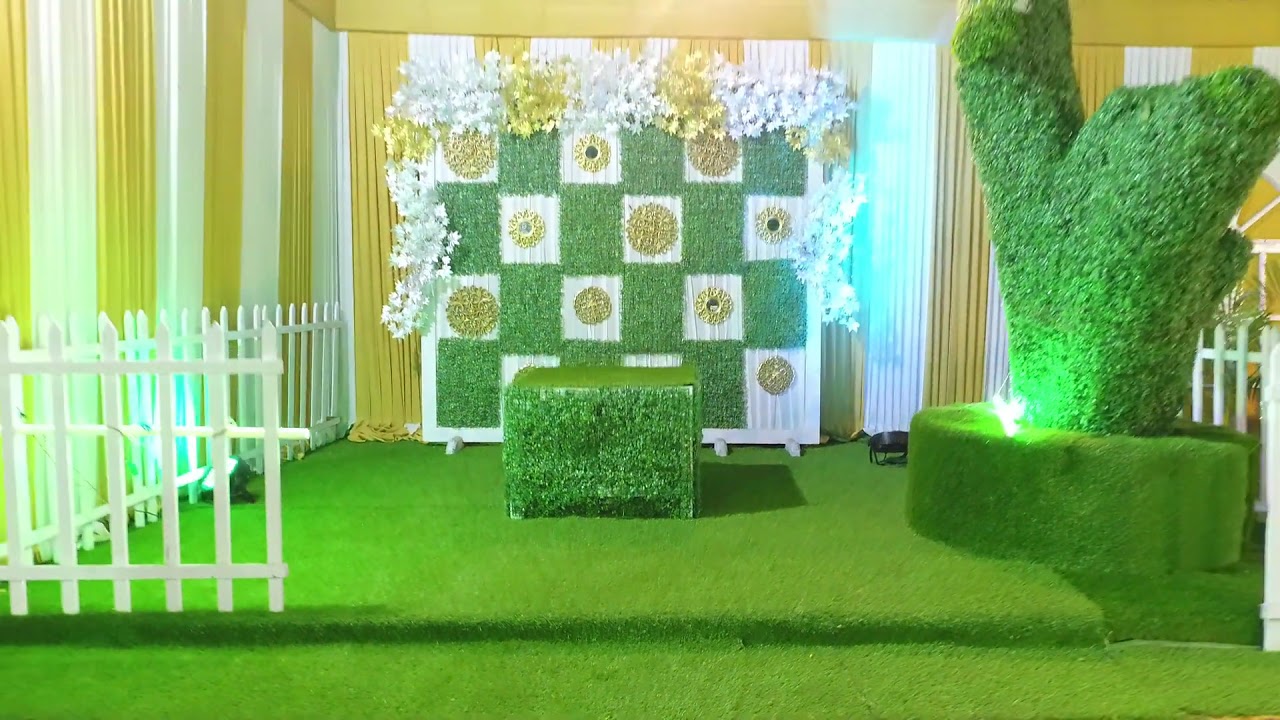The image features an intricately designed indoor setting that mimics an outdoor garden scene, with synthetic materials used throughout. The floor is covered in a green grass turf, giving an appearance of a lush, manicured lawn. A small platform, also covered in the same green turf, can be accessed via a slight step up and is bordered by a pristine white picket fence.

At the forefront on the right side, there is an artificial tree stump adorned with green leaves, set on a round base, designed to appear as if it is growing from the platform. The backdrop is dominated by a checkerboard pattern composed of alternating green and white squares. Each white square features a gold circle in its center, adding a touch of elegance. The entire checkerboard is framed with a trim that appears to be made of white and gold flowers or confetti, enhancing the thematic decor.

Curtains border the scene, alternating between white and gold, contributing to the overall cohesive, vibrant look of the setting. The bright and clear lighting illuminates the space, indicating that the scene is likely intended for photo opportunities, possibly for an event with a spring or garden theme. The combination of elements creates a whimsical, picturesque environment that feels both festive and meticulously crafted.